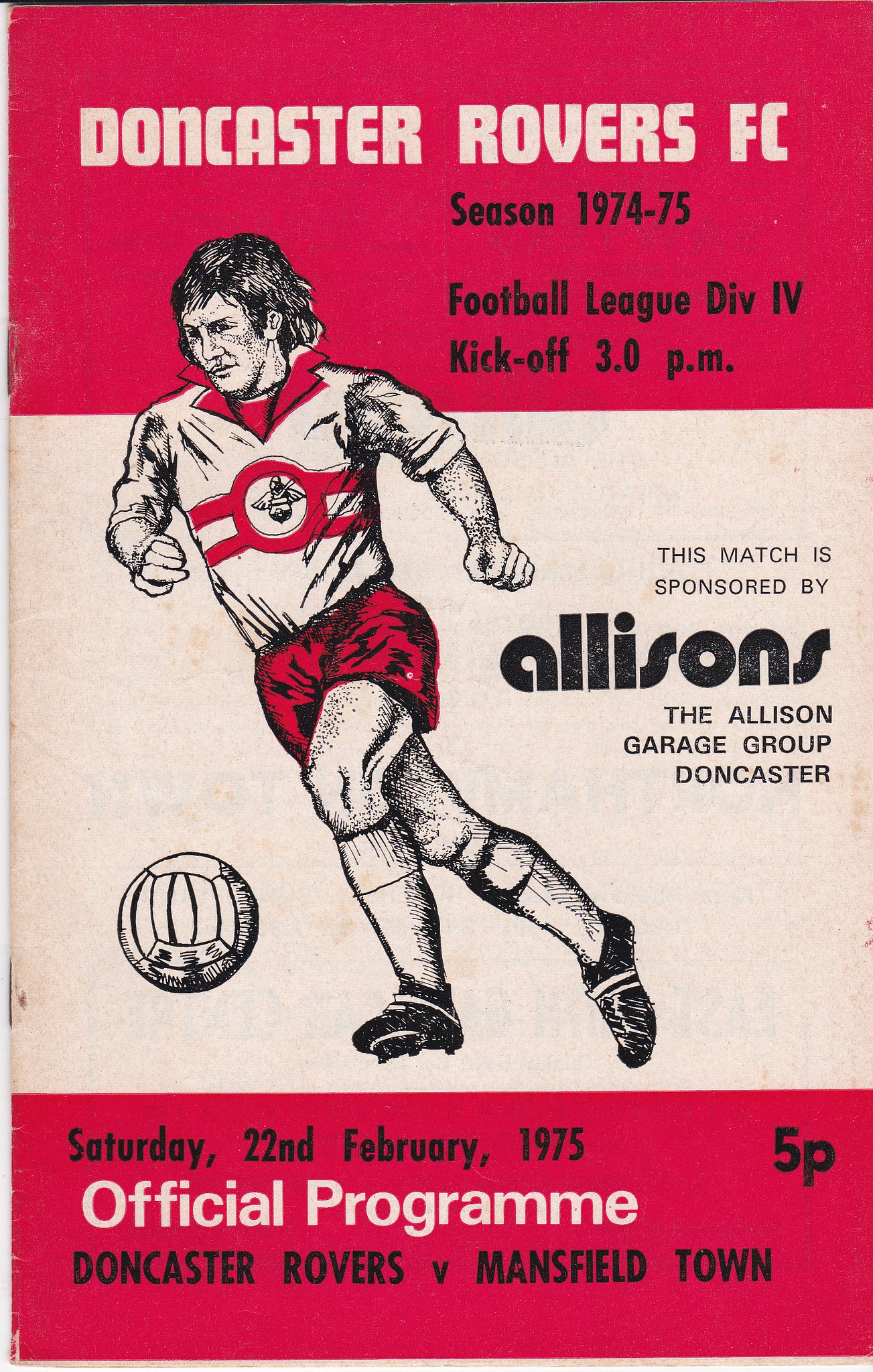This image is of an official soccer program for a match between Doncaster Rovers and Mansfield Town. The layout features a prominent white and red color scheme, with detailed text and graphics. At the top, on a red background, it reads "DONCASTER ROVERS FC" in bold white letters. Beneath it, in black text, it states, "Season 1974-75, Football League Division 4, Kickoff 3 p.m." The central portion of the program shows a black and white drawing of a soccer player in a red and white jersey with red shorts, captured mid-action as he kicks a soccer ball. To the right of this illustration, there is a note that reads, "This match is sponsored by Allison’s, the Allison Garage Group, Doncaster." At the bottom, another red bar contains additional important details: in white text, it says "Official Program" and "Doncaster Rovers vs. Mansfield Town," alongside the date "Saturday, 22 February 1975," and "5p." The detailed design and layout emphasize the importance and formality of this Division 4 match.